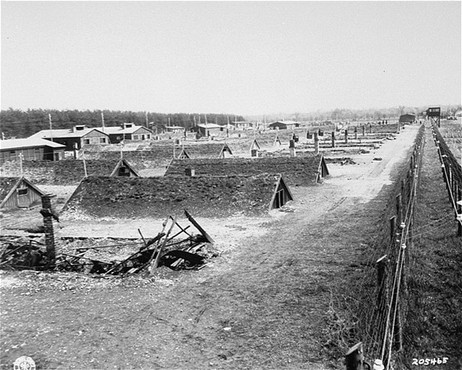This black-and-white photograph, dated by the number 205465 in the bottom right corner, captures a stark and desolate scene that seems reminiscent of a mid-20th century landscape, possibly associated with a prison or work camp. The image features a row of dilapidated A-frame structures, most of which are low to the ground, with just their raised roofs visible above the earth. The first building in the foreground is in ruins, with only a chimney standing amidst the collapse of its wooden roof. Further back, two more complete A-frame barracks emerge, their doors or shutters partially visible. Stretching into the horizon, additional rows of these structures are discernible, though their details blur in the distance. On the right side of the photo, a long fence runs almost the entire length of the image, cutting across the clear sky and empty landscape. The photograph captures a somber and neglected array of buildings, set against a backdrop that evokes a feeling of isolation and wear.